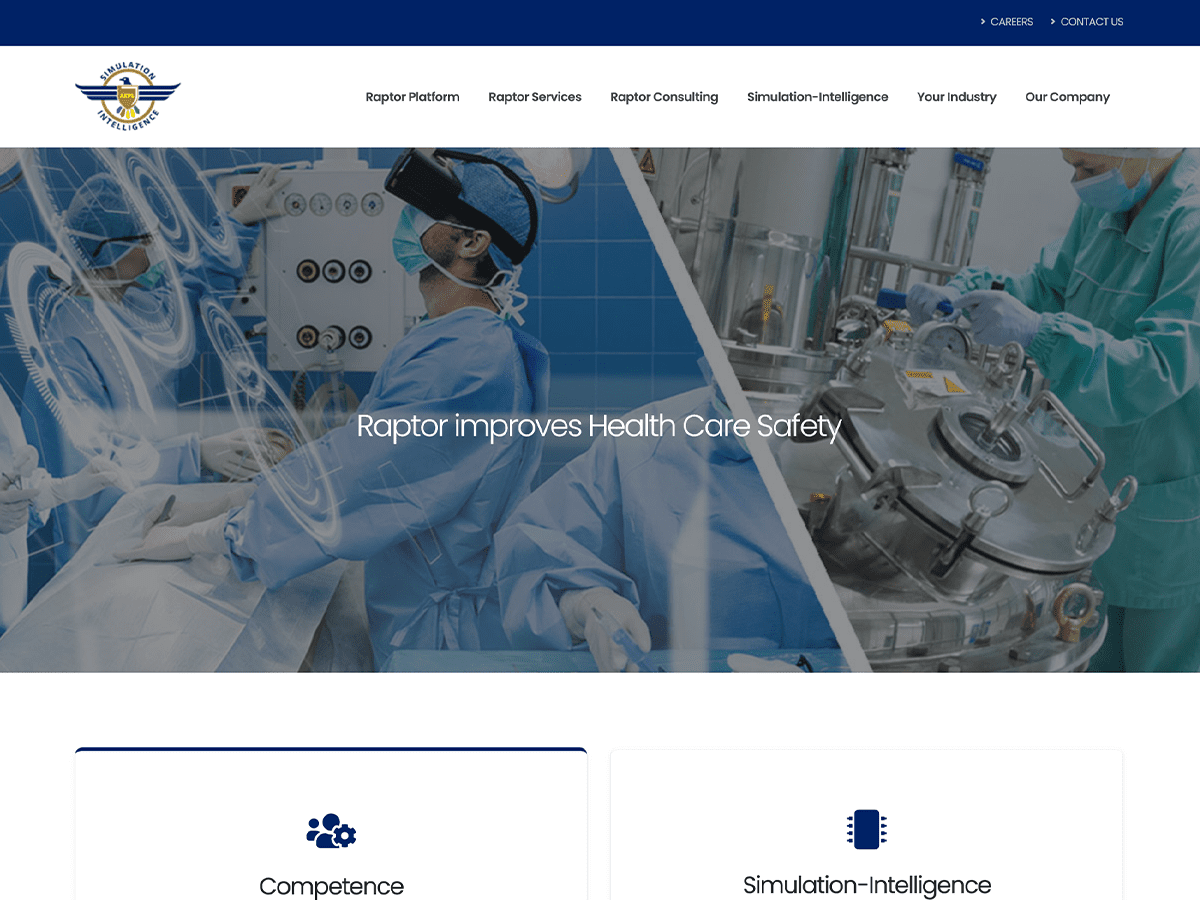In this detailed image, we observe a sophisticated 3D or virtual reality (VR) interface designed to aid in surgical procedures. In the top left corner, there is an icon of a raptor accompanied by the words "Simulator Intelligences," with "Simulator" above the raptor and "Intelligences" below. Directly under this, six clickable options are displayed: "Raptor Platform," "Raptor Services," "Raptor Consulting," "Simulation Intelligence," "Your Industry," and "Our Company."

In the top right corner, there are additional clickable options labeled "Contact Us" and "Careers." Central to the image, a surgeon equipped with VR goggles is depicted performing a surgical procedure. Adjacent to this, on the right, a medical device is illustrated. Both of these images are overlaid with the text, "Raptor Improves Healthcare Safety," in bold white letters.

Beneath these images, there are clickable areas marked by the symbol and word "Competence," as well as "Simulation Intelligence." This detailed arrangement highlights the advanced capabilities and resources provided by the Raptor platform to enhance the safety and efficiency of healthcare practices through simulation technology.